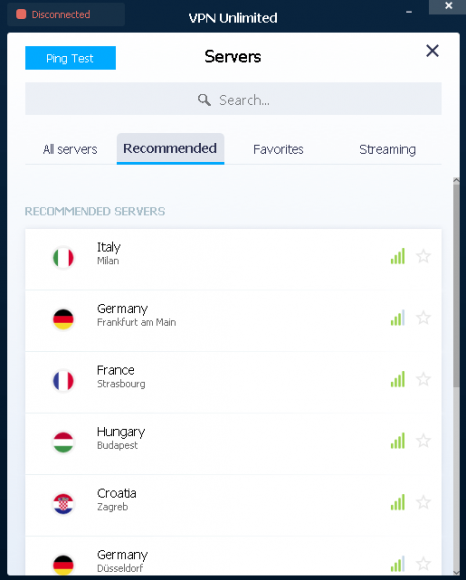The image is a screenshot from a cell phone displaying a VPN application interface. In the upper left-hand corner, the word "Disconnected" is prominently shown in red letters. Adjacent to this, there is a label that reads "VPN Unlimited". Below this, the phrase "Ping Test" appears in blue, indicating a feature that can be used to run a connectivity test. To the right, the word "Servers" is displayed in black text.

Further down the screen, there is a search bar with a magnifying glass icon accompanied by the placeholder text "Search...". Continuing downward, there is a section labeled "All Servers", followed by "Recommended", which has a blue underline indicating it is the current selection. Other tabs labeled "Favorites" and "Streaming" are also visible.

In the "Recommended Servers" section, a list of countries is displayed. Each country's name is accompanied by its national flag on the left side. On the right side, there is a blank space followed by three green bars resembling a signal strength indicator. Next to these bars, there are faint gray stars suggesting user interaction for marking favorites. The countries listed from top to bottom are Italy (Milan), Germany, France, Hungary, Croatia, and another entry for Germany at the bottom.